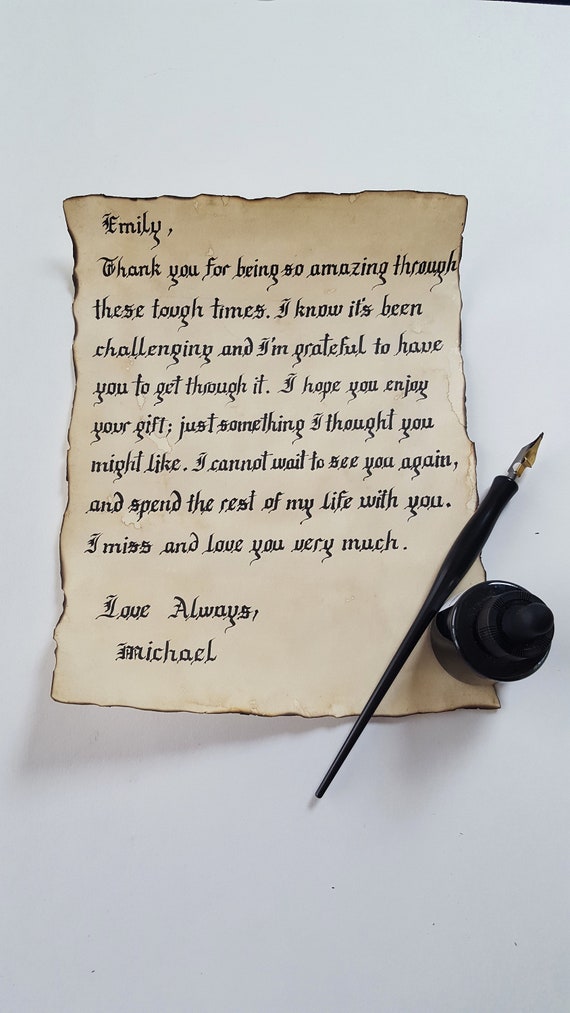The image is an intricate illustration featuring a heartfelt letter on a piece of parchment-like paper with burnt, irregular edges, giving it an antique and somewhat mystical appearance. The parchment, positioned against an off-white or very light gray background, is inscribed in an old-English script. The letter reads: 

"Emily, thank you for being so amazing through these tough times. I know it's been challenging, and I'm grateful to have you to get through it. I hope you enjoy your gift, just something I thought you might like. I cannot wait to see you again and spend the rest of my life with you. I miss and love you very much. Love always, Michael."

On the bottom right corner of the note lies a vintage quill-tipped pen, with the pen’s tip extending beyond the paper, alluding to its use in crafting the letter. Beside the pen, there is an ink bottle with a black cap, emphasizing the traditional writing method portrayed in the image. The scene is rendered with such realism that it teeters between looking like an actual photograph and a meticulously detailed computer-generated illustration.